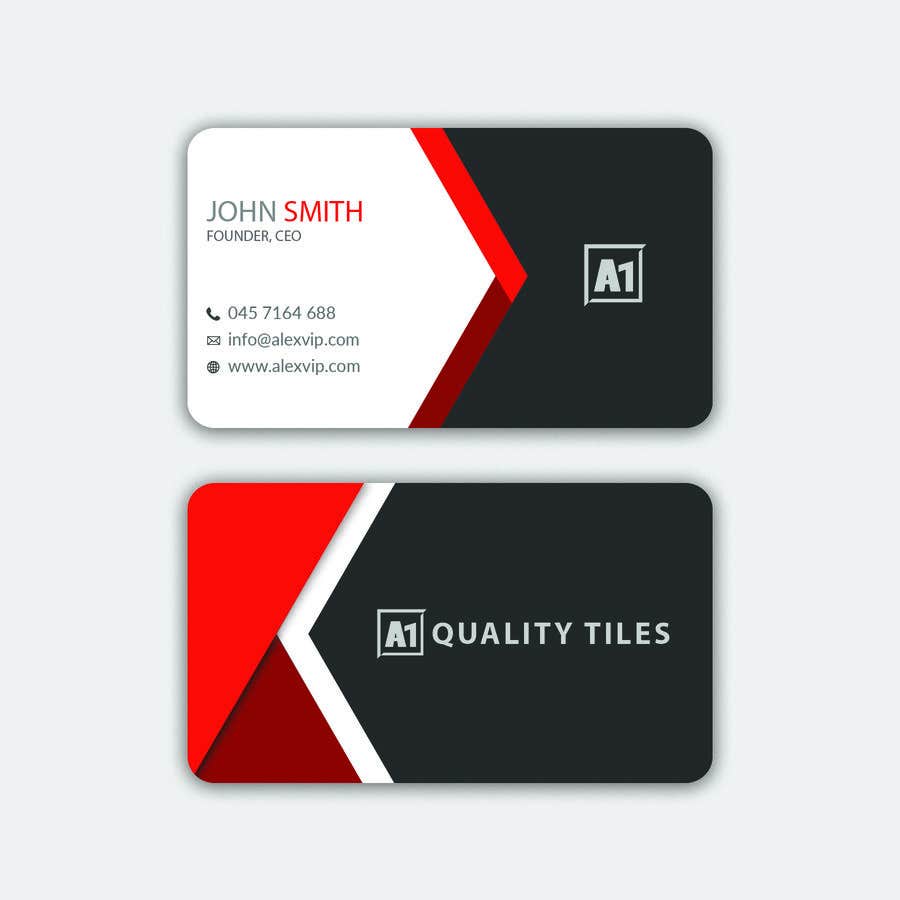The image features a digital rendering of a business card set against a light gray background. The cards are displayed vertically with the front of the card on top and the back on the bottom. Both cards are rectangular with rounded corners.

The front of the card has a white left section bordered by a narrow red strip, and a black right section. On the white section, "John" is written in gray and "Smith" in red, followed by "Founder, CEO" in smaller gray text. Below his designation, there's a telephone icon with the number "045-716-4688," a mail icon, and an email address "info@alexvip.com." The black section features a centered gray frame encompassing block letters "A1."

The back of the card mirrors the structure but with a red left section and a white border leading into the black right section. This time, the black section prominently displays "A1 Quality Tiles" in a similar gray framed style.

The meticulous design uses a color palette of white, red, black, and gray, ensuring clarity and visual appeal while delivering essential contact information and brand identity. Shadows around the cards on the gray background add depth to the digital rendering.